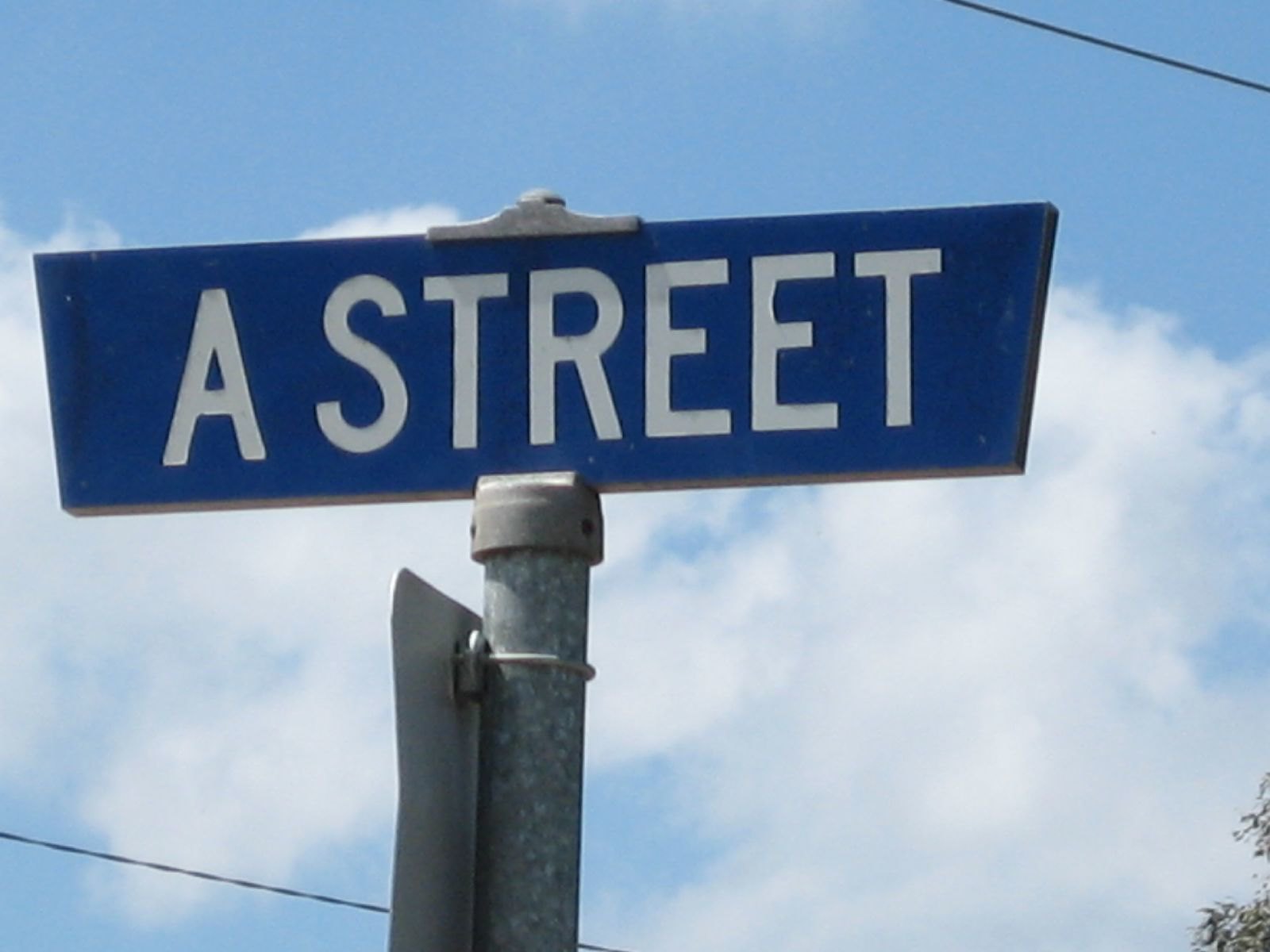The image captures a scene with a clear blue sky, interspersed with wisps of white clouds concentrated towards the bottom. The vibrant blue patches are visible even through the cloudy sections, adding a picturesque contrast. Prominently featured is a gray metal post extending vertically, supporting a distinct blue sign. This sign, shaped like a parallelogram, is secured by silver brackets at its top and bottom. Printed in bold white letters, the sign reads "A Street." Additionally, a thin silver wire connects to another sign positioned in the opposite direction, revealing only its silvery back without any visible text.